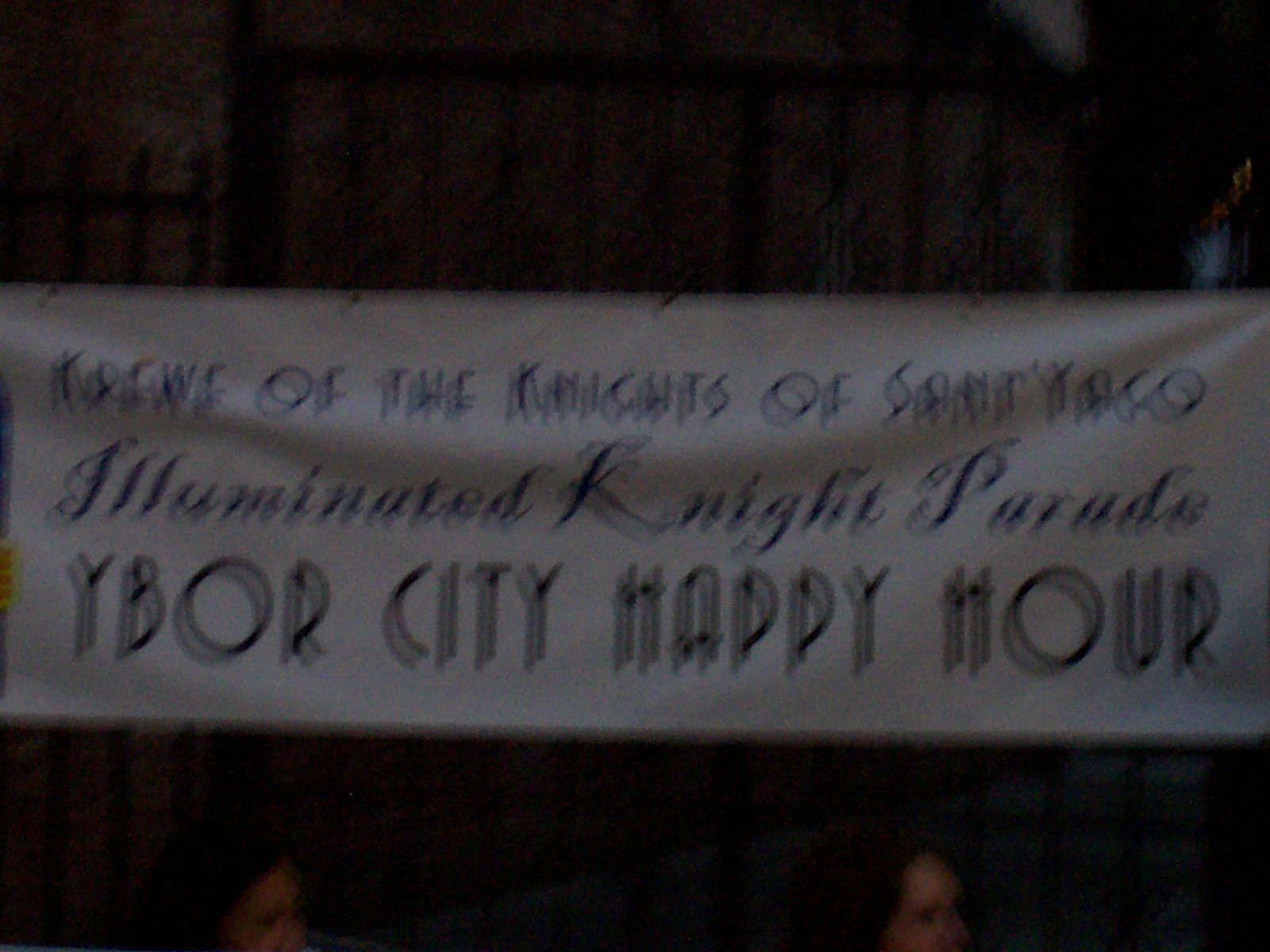In the center of this image with a dark background, a prominent white banner spans across more than one third of the total space. The banner captures attention with its elegant, albeit somewhat hard-to-read, script. Positioned at the top of the banner, in a graceful italic script, it reads: "Illuminated Our Night Parade." Below that, in bold, flowing script, the main inscription says, "Wybor City Happy Hour." At the very top, slightly more difficult to decipher, is another phrase suggesting, "Nights of Sanpico" or a similar name related to an event, adding to the mysterious allure of the parade announcement.